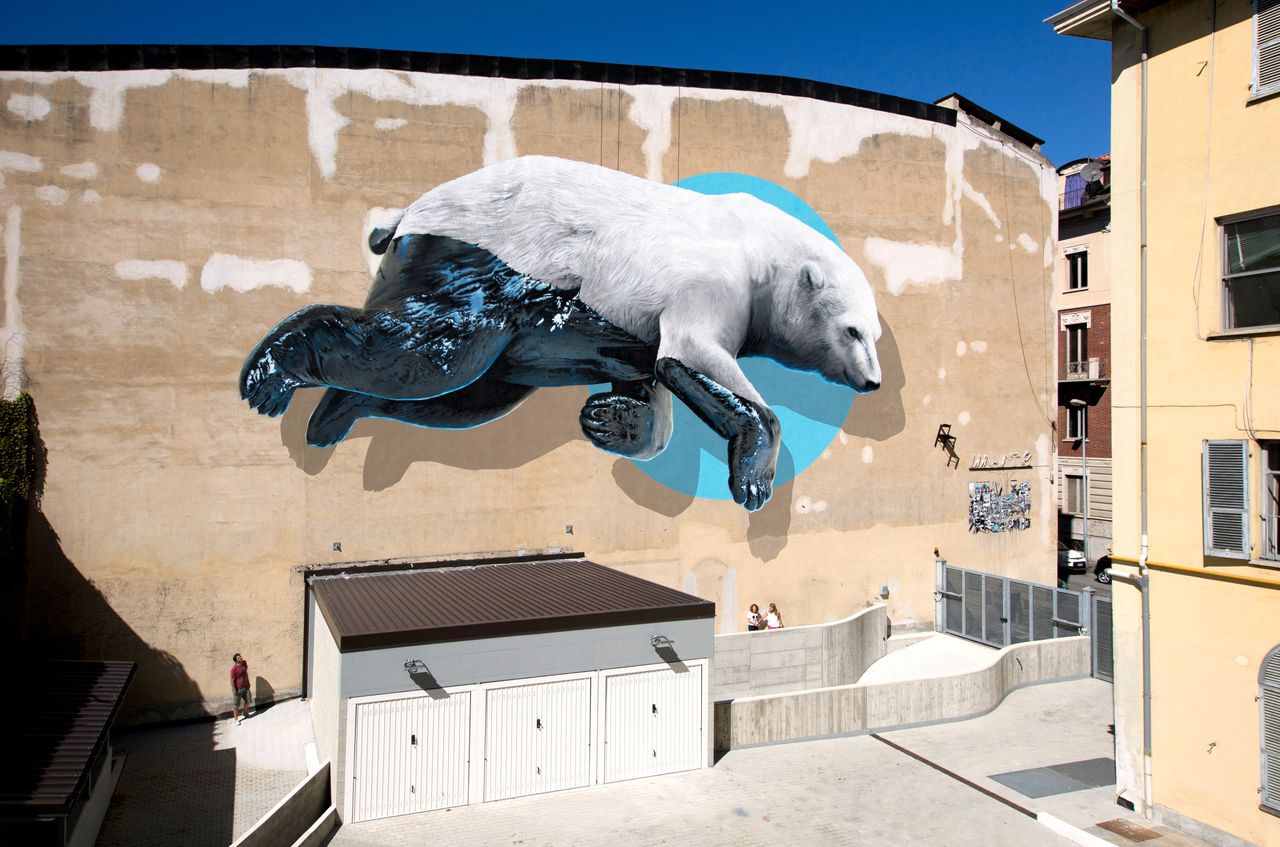The photograph captures a large, detailed mural of a polar bear on the side of a tan and white colored building overlooking a city parking lot. The polar bear, depicted with a realistic and striking appearance, appears to be swimming in the air. Its top half is white, while the bottom half is smeared with slick, black oil, possibly conveying a message about pollution. A round blue circle forms a backdrop behind the bear's head, enhancing its striking presence. Below the mural, the building features three garage doors and is surrounded by a light gray asphalt parking lot. In the scene, a solid gray metal fence, likely automatic, closes off the parking area. Adjacent to this building is a multi-story residential structure, also in a tan color. Three people are scattered around the lot; one on the left side with his shadow cast on the wall, and two on the right side near the garage doors.